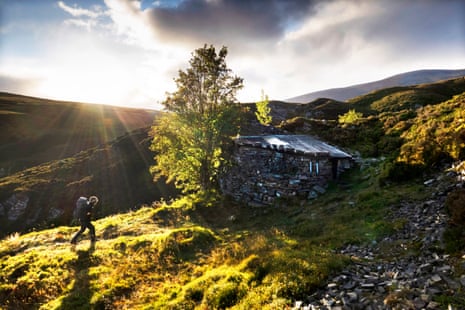In this slightly blurry, landscape-oriented photograph, an idyllic countryside scene unfolds. Dominating the center of the image is a very old stone cabin, constructed on a gently sloping grassy hillside adorned with light green grass. To the immediate foreground on the left, a solitary, towering tree stands, its height almost twice that of the cabin beside it. A hiker, clad in black and carrying a sizable backpack, is captured walking towards the stone structure from the bottom left corner of the image.

The hilly terrain incorporates varied elements including a stacked array of grayish rocks towards the bottom right corner. Further in the distance, the landscape continues to roll into higher hills and mountainous ranges. The sky above is mostly cloud-laden, especially in the top right, while a vibrant sun peeks out from behind a mountain ridge, casting radiant sunbeams that illuminate the entire scene and create long shadows over the terrain. This creates a striking contrast against the partly cloudy sky, enhancing the rustic, serene atmosphere of the countryside setting.